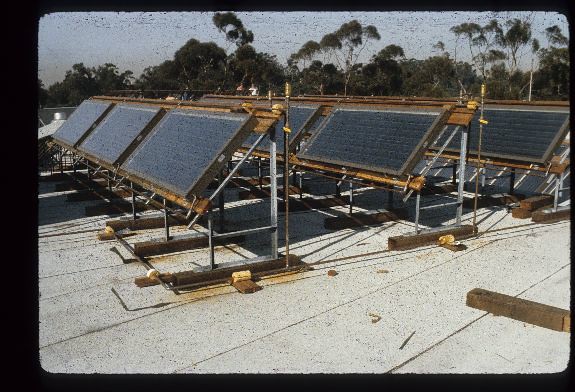The photograph is a rather faded color image taken outdoors during daytime, capturing the roof of a building covered in solar panels. The panels, arranged in three visible rows, total to eight and are set on rusty metal bars, which are also supported by rusty poles. The roof appears to be made of gray rolled roofing, possibly tar or cement. The horizon reveals treetops and a patch of blue sky. In the far right corner, there is a solitary piece of wood, roughly the size of a 2x4. The photo, framed by a black border, suggests an older era, with the central focus on the solar panels themselves, which are centered and angled towards the sky. The overall quality of the photograph is unclear, adding to the aged appearance of the scene.